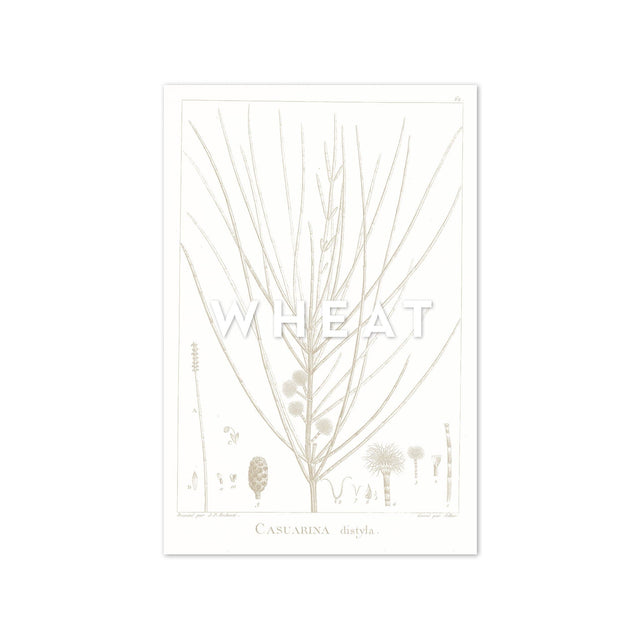The image portrays a detailed botanical illustration on a white background with a white border framed by dark lines. Central to the composition is a prominent plant with slender branches and stems, identified as a wheat plant. The main plant features some leaves in the lower middle section, and it's accompanied by smaller illustrations on either side that likely represent different stages of the wheat plant's lifecycle. The upper portion of the image has the word "WHEAT" in capital block letters, subtly highlighted by shadows against the white background, making it slightly difficult to discern at first glance. Below the central plant, there are additional plant-like drawings, including elements resembling a pine cone and small flowers. At the very bottom of the image, the words "CASUARINA DISTYLA" are written, perhaps indicating the plant species or related information.